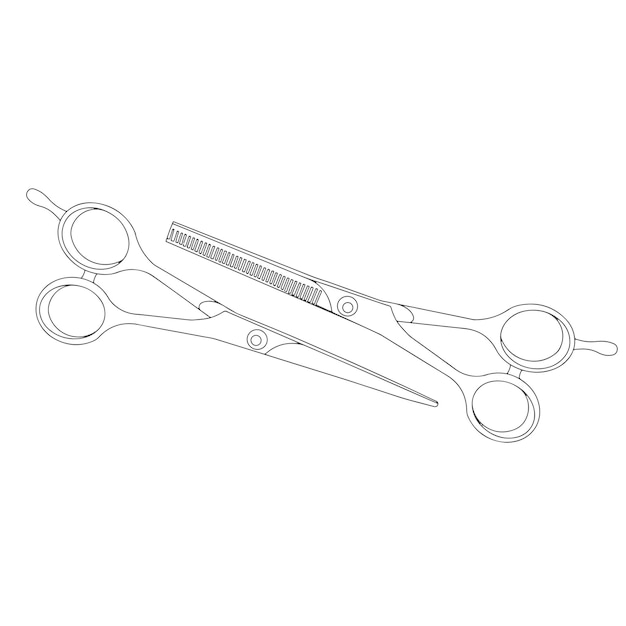The image is a computer-generated, cartoon-like outline drawing of two pairs of scissors commonly used by barbers, set against a white background. Both pairs are depicted in black ink, resembling a sketch made with a black pen or pencil. The scissors feature handles, one pair positioned on the left side with the blades facing right, and the other on the right side with the blades facing left, creating a mirrored arrangement.

One pair of scissors, likely used for standard hair cutting, has sharp, pointy blades at the ends. The other pair, designed for thinning hair, has a texturizing blade shaped like a comb with flat ends. Both scissors possess the typical thumb and finger holes for gripping, with a protruding knob-like feature on the top hole of each pair. A small nut or bolt situated in the center of both pairs allows the blades to pivot. The image has no background elements or text, focusing solely on the outlined form of the scissors.